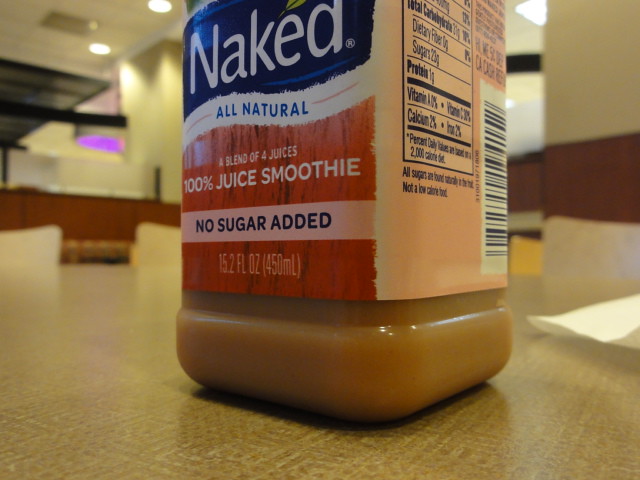This meticulously detailed close-up color photograph captures the bottom half of a Naked Juice smoothie bottle placed on a mustard-colored, patterned Formica countertop. The bottle, appearing square with rounded edges, showcases a series of colorful and prominent labels. Starting from the top, the brand name "Naked" is displayed in bold white letters on a dark blue background. Beneath it, a white band with blue text reads "All Natural," flanked by small red vertical lines. Following this, a red strip with subtle black vertical lines holds the phrase "100% Juice Smoothie" in white. Directly under this, a pink strip features the message "No Sugar Added" in blue font. Towards the bottom, on a white section of the label encased in red, it states "15.2 fluid ounces (450 milliliters)." The juice itself is a murky brownish-orange hue, and only the front and part of the side of the bottle are visible, with the nutritional facts and barcode in a dark font on a peach background. In the surrounding environment, the mustard yellow-patterned countertop is prominent, and there is a glimpse of a white ceiling with overhead lights and a mustard-colored wall in the upper left corner of the image. Additionally, there appears to be part of a sheet of paper or napkin on the right side of the table.